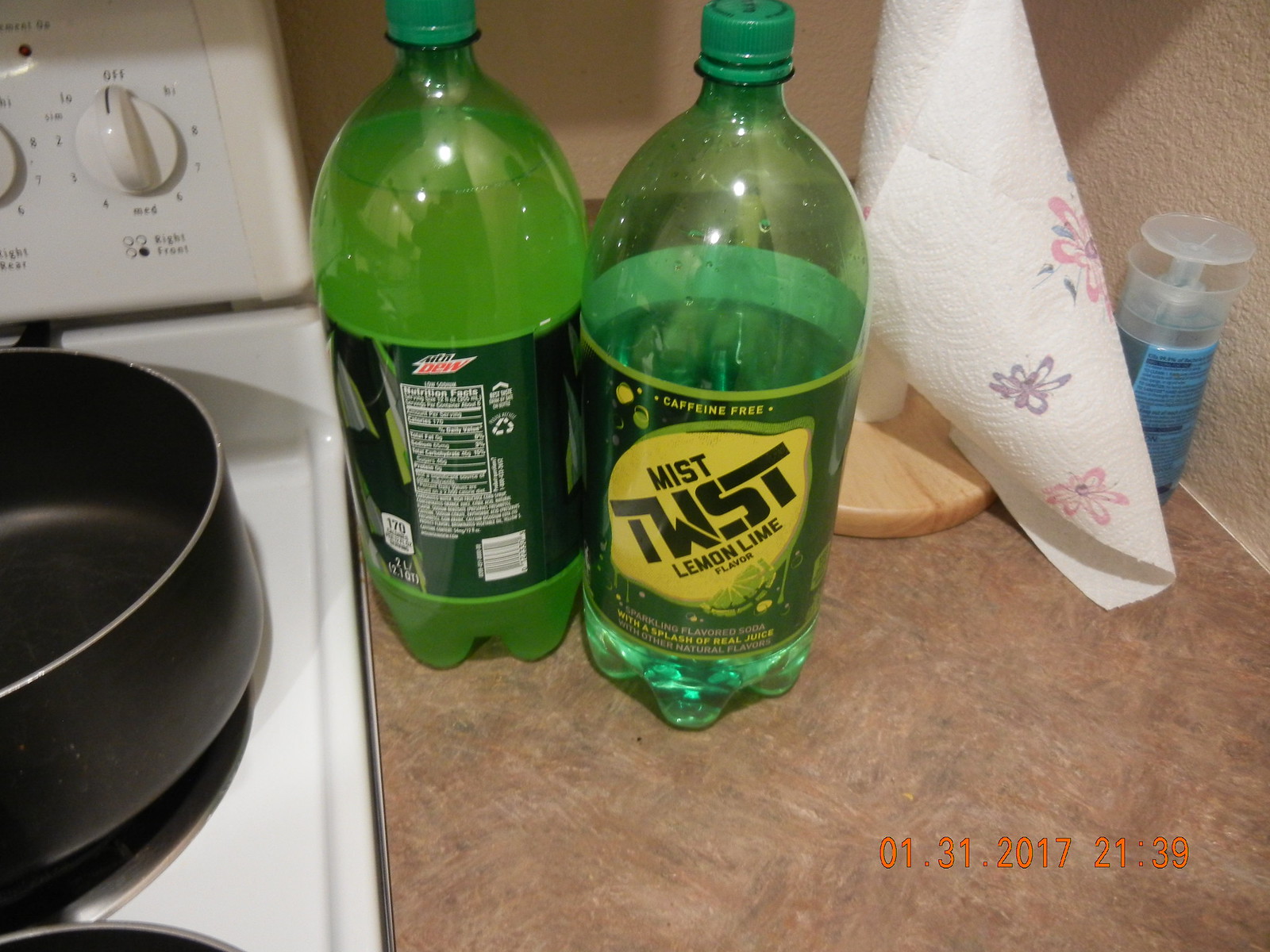This color photograph captures the interior of a kitchen with a brownstone countertop prominently displayed on the right side. The image is timestamped with orange numbers at the bottom: "01-31.2017" at "21:39". On the countertop, there are two bottles of soft drinks - one is half-filled with Mist Twist Lemon Lime Soda, exhibiting a clear greenish color, and the other is a full, unopened bottle of Mountain Dew, which appears cloudier. Additionally, a roll of paper towels is placed on the counter. To the left, a white stove with a black pan on the stovetop is visible, adding to the everyday domestic scene captured in this photograph.